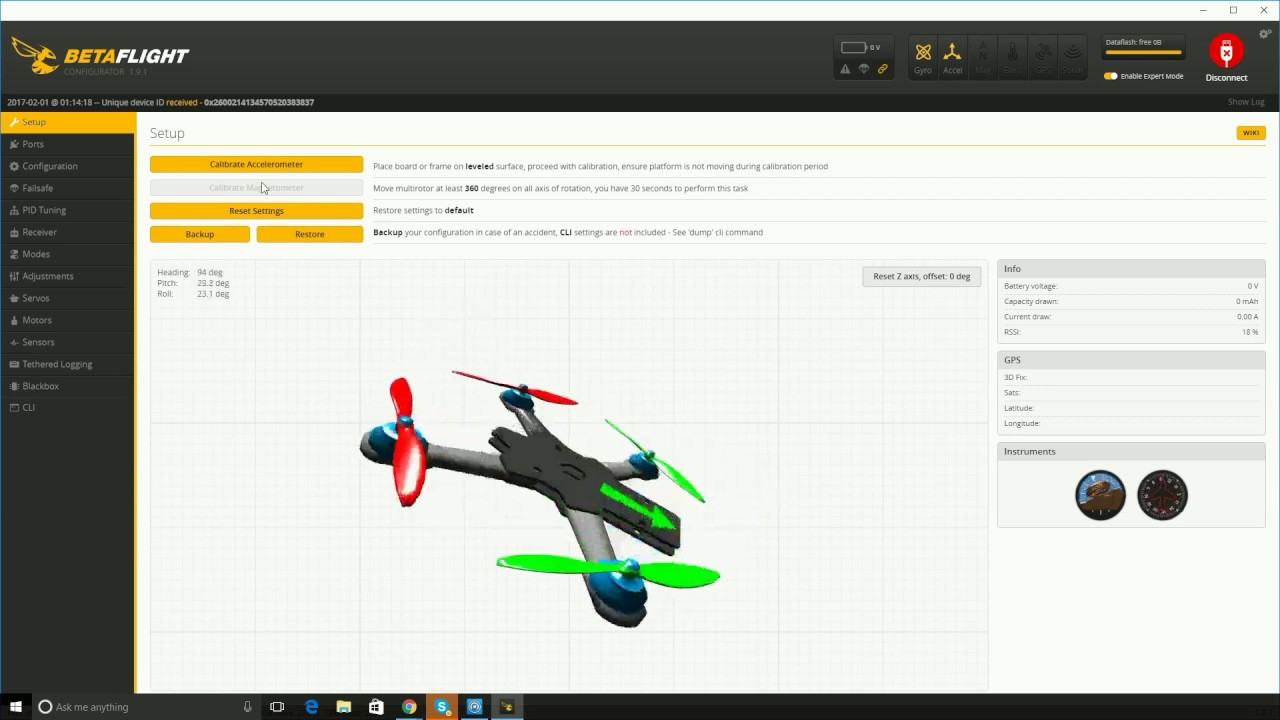This screenshot captures a section of a website, seamlessly identified by the "Betaflight" logo situated in the top left-hand corner. The logo exhibits the word "Beta" in yellow and "flight" in white. To the left of the screen, there is a vertical menu comprising various clickable options. The website interface employs a light mode, characterized by its predominantly white background.

Dominating the center of the webpage is a detailed image of a flying drone. The drone, styled in striking black and white, adopts an X-shaped design, featuring four propellers. The propellers are vividly color-coded, with two in light green and the other two in red. Centrally, between the two green propellers, a green arrow directs the viewer's attention diagonally towards the bottom right-hand corner of the image.

At the bottom of the screen, a visible taskbar reveals that this screenshot was captured on a Windows operating system. The taskbar includes a prominently positioned white Windows key in the bottom left corner. Multiple application icons are displayed, offering quick access to frequently used programs like the Chrome browser, Internet Explorer, Windows Store, and File Manager.